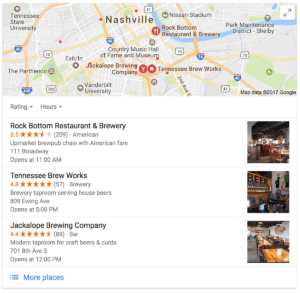The image features a map of Nashville, Tennessee, set against a white background with thin blue lines framing the edges. At the top of the image, the map includes several red pins marking specific locations. Below the map, there's a detailed listing of breweries in the area, each accompanied by their respective ratings and pictures. 

1. **Rock Bottom Restaurant and Brewery**:
   - **Rating**: Approximately 3.5 stars
   - **Image**: Positioned to the right, depicting the establishment.

2. **Tennessee Brew Works**:
   - **Rating**: 4.5 stars
   - **Image**: Also placed to the right, showing the venue.

3. **Jackalope Brewing Company**:
   - **Rating**: 4.4 stars
   - **Image**: Positioned to the left, offering a glimpse of the location.

Below these listings, there's a small blue box with the text "more places," indicating additional recommendations.